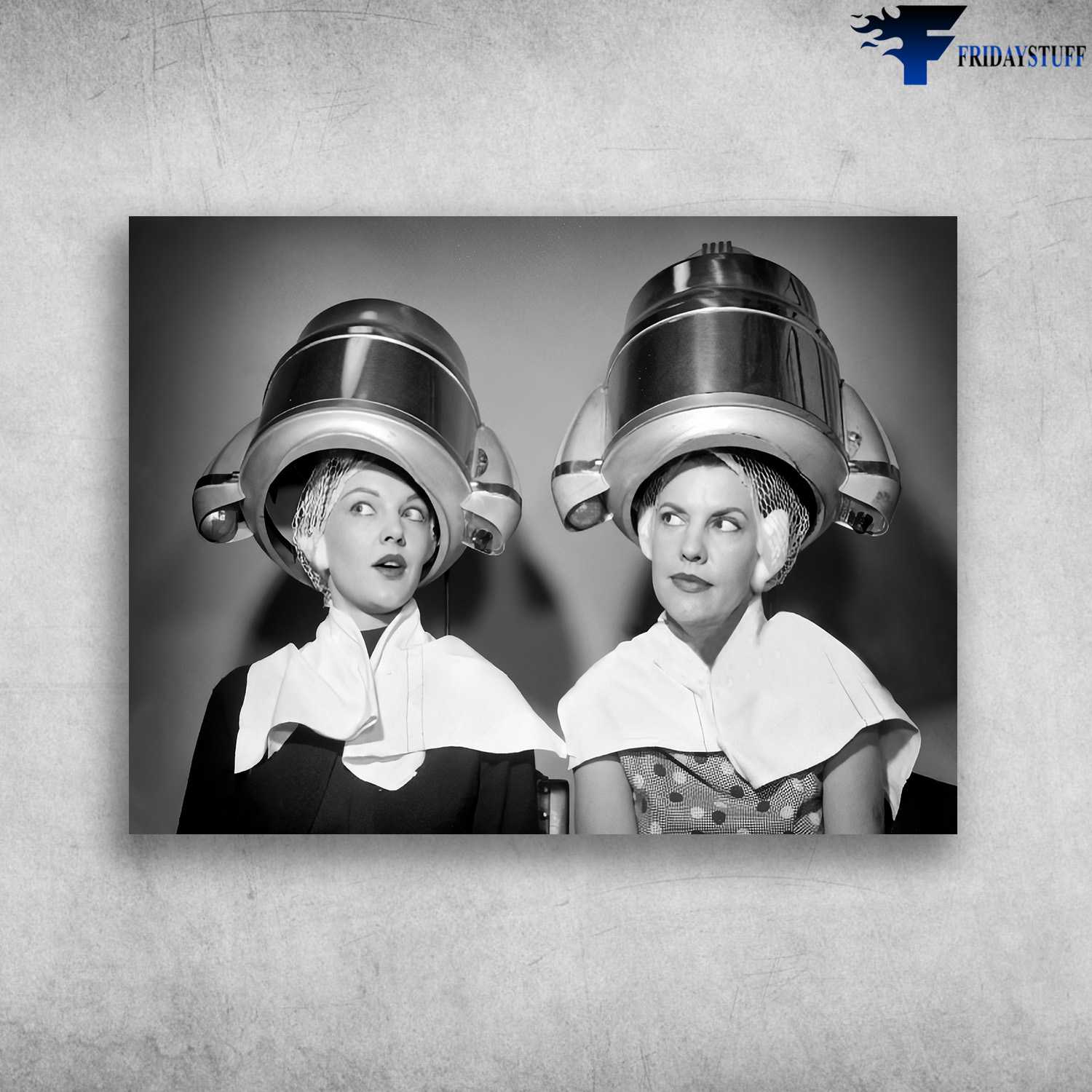This black and white photo, set against a light gray matted backdrop, features two women sitting under shiny silver, old-fashioned hair dryers that are mounted on the wall. Both women, with their hair wrapped in curlers and netting, have white towels draped over their shoulders to protect their clothing. The woman on the left is dressed in a dark outfit, likely a black sweater, and is gazing upwards to the left with her mouth open, as if talking. The woman on the right, attired in a polka-dotted dress, is similarly looking towards the left, appearing engaged in the conversation. Their ears are protected with cotton balls, suggesting they are in a mid-20th century beauty salon, probably from the early 1950s to 1960s. The photo conveys a moment of shared gossip or friendly chat while getting their hair done. The top edge of the image's matting features the words "Friday Stuff," adorned with black and blue lettering and flames, adding a thematic touch to the vintage scene.